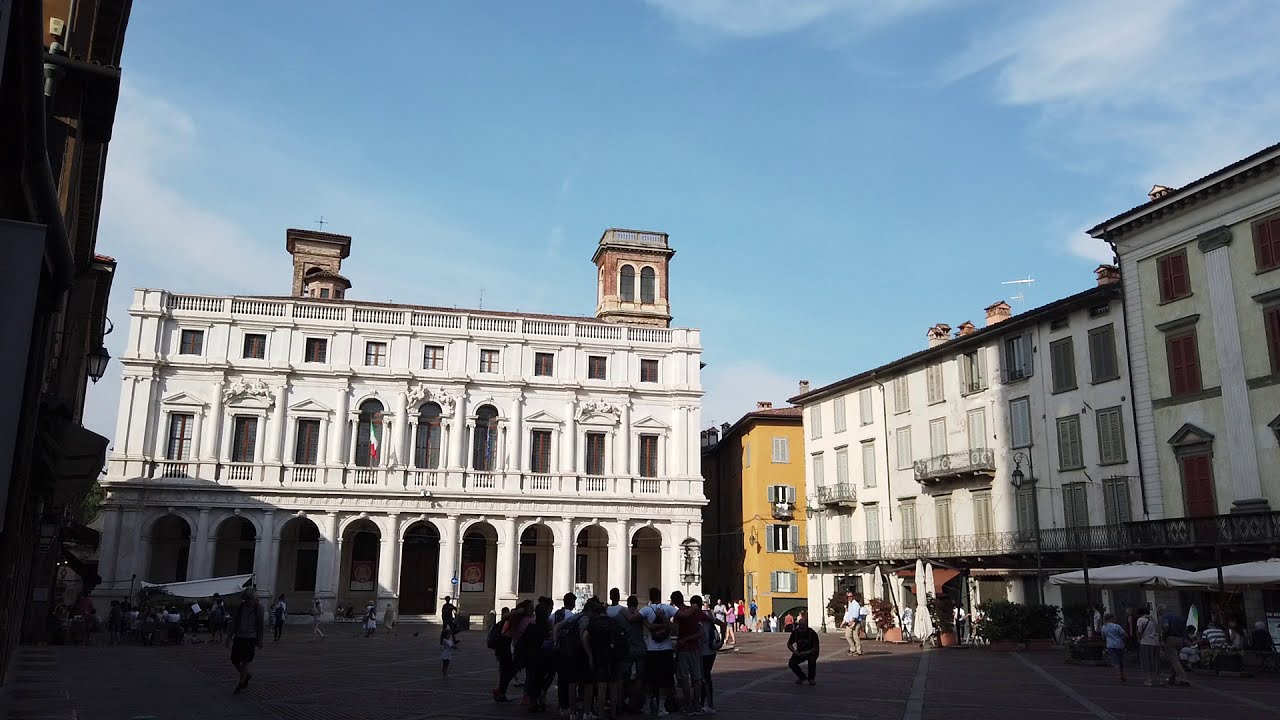In the photograph, taken outside during the daytime in a wide city square, we find ourselves standing in the shadow of a very tall building on the left-hand side. At the center bottom of the image, a group of people is huddled in a circle or semi-circle, appearing like tourists engaged in conversation. To their right, a man is crouched down, seemingly ready to take a picture of the group.

The image prominently features a large, white, three-story historical building occupying the background. The building's ground level showcases tall arched columns as entrances. The second story has a mix of arched and narrow rectangular windows, some adorned with decorative carvings and stone balconies, while the top floor features smaller rectangular windows. A green, white, and red flag, believed to be Italian, hangs from the second level, adding a European ambiance to the scene. There is also a blue flag visible on the building.

To the right side of this main building, there is another significant white structure characterized by wrought-iron railings and European architectural elements. Between these two buildings, a mustard-yellow building adds a splash of color, while farther to the right, a smaller pale-yellow building is noticeable. Above these buildings, the sky is bright blue with wisps of white clouds, enhancing the picturesque setting. The square below bustles with many people moving to and fro, contributing to the lively atmosphere of this European city square.